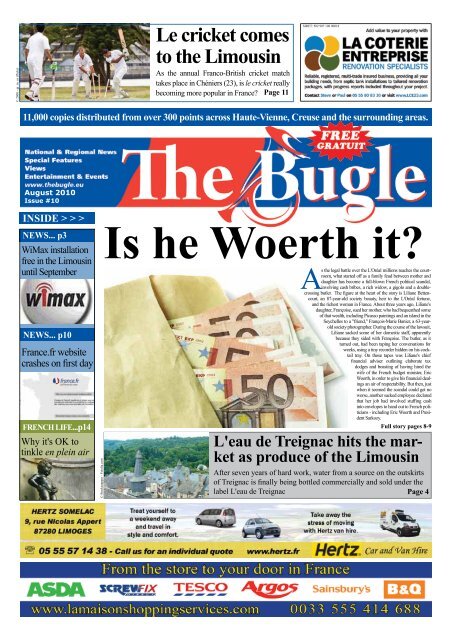The front page of the French newspaper, The Bugle, dated August 2010, features a prominent title in white text set against a blue-red-blue background with a bold "FREE" in red adjacent to it. In the upper left corner, a photograph of three men dressed in white uniforms playing cricket is captioned with "Le Cricket Comes to Limousin." Beneath the title, an article titled "Is He Worth It?" is accompanied by an image of an envelope stuffed with $50 bills. Another article below this reads "Loudy Trinak Hits the Market as a Produce of the Limousine," likely discussing regional agricultural products. The bottom section of the page includes ads for car rentals, including Hertz, and several logos from major stores such as ASDA, Tesco, Argos, B&Q, and Sainsbury’s, with the slogan "From the Store to Your Door in France." The newspaper's website is listed as www.thebugle.au or .eu, and it is issue number 10.